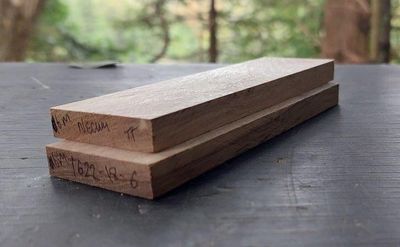The photograph captures a close-up view of two rectangular pieces of pre-cut lumber, likely 1x4s and approximately 12 to 14 inches long, stacked diagonally from the bottom left to the top right on a dark gray or black wooden table. The table appears to be placed outdoors, as the background features blurred tree trunks, greenery, and hints of brown, suggesting a natural setting. The ends of the lumber facing the camera have handwritten text and numbers, possibly in pencil. The top piece appears to have "NECURY T T" and "6M," while the bottom piece shows "2622-18-6" and "6M," though the text is somewhat difficult to decipher.